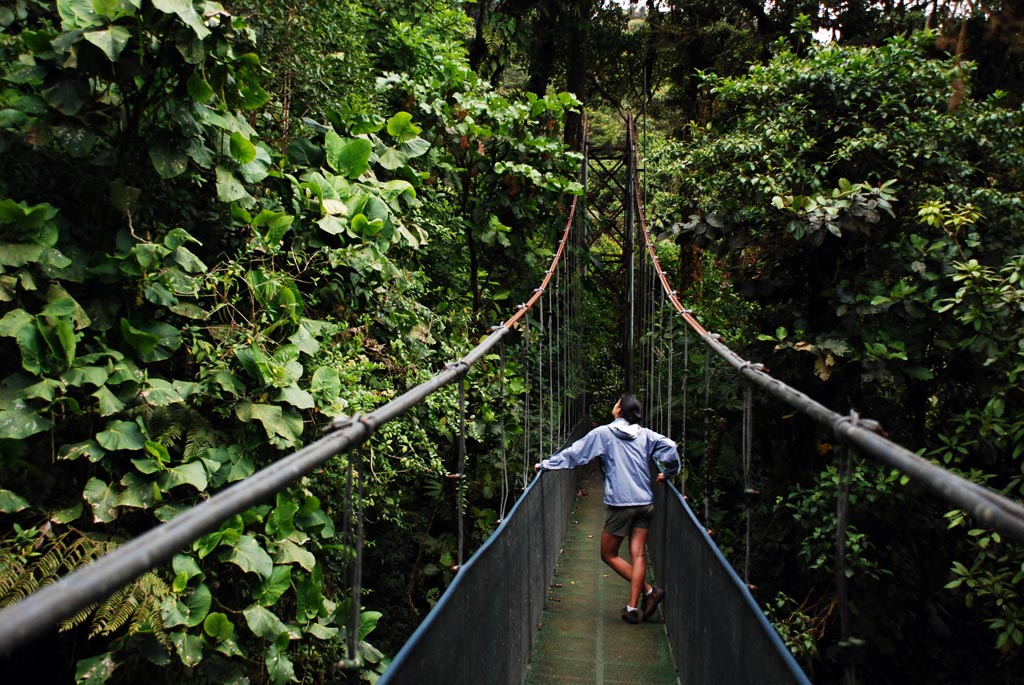In this captivating photograph, we see a dense jungle forest teeming with lush greenery and vibrant foliage. A long, narrow suspension bridge, featuring black to bronze railings, cuts through the center of the image, suspended high above a deep drop. The bridge itself has a greenish-brown hue. At the forefront stands a woman with lightly tanned skin, clad in a light blue anorak-style windbreaker, shorts, and hiking shoes. Her dark black hair is neatly pulled back into a bun. She is captured in a moment of contemplation, looking up toward the verdant canopy. Her left hand grips the railing on her side while her right hand reaches across to the opposite railing. With one leg bent and crossed over the other, her posture adds a sense of serene balance as she gazes upward into the surrounding greenery. The scene exudes a sense of tranquility and connection with nature.